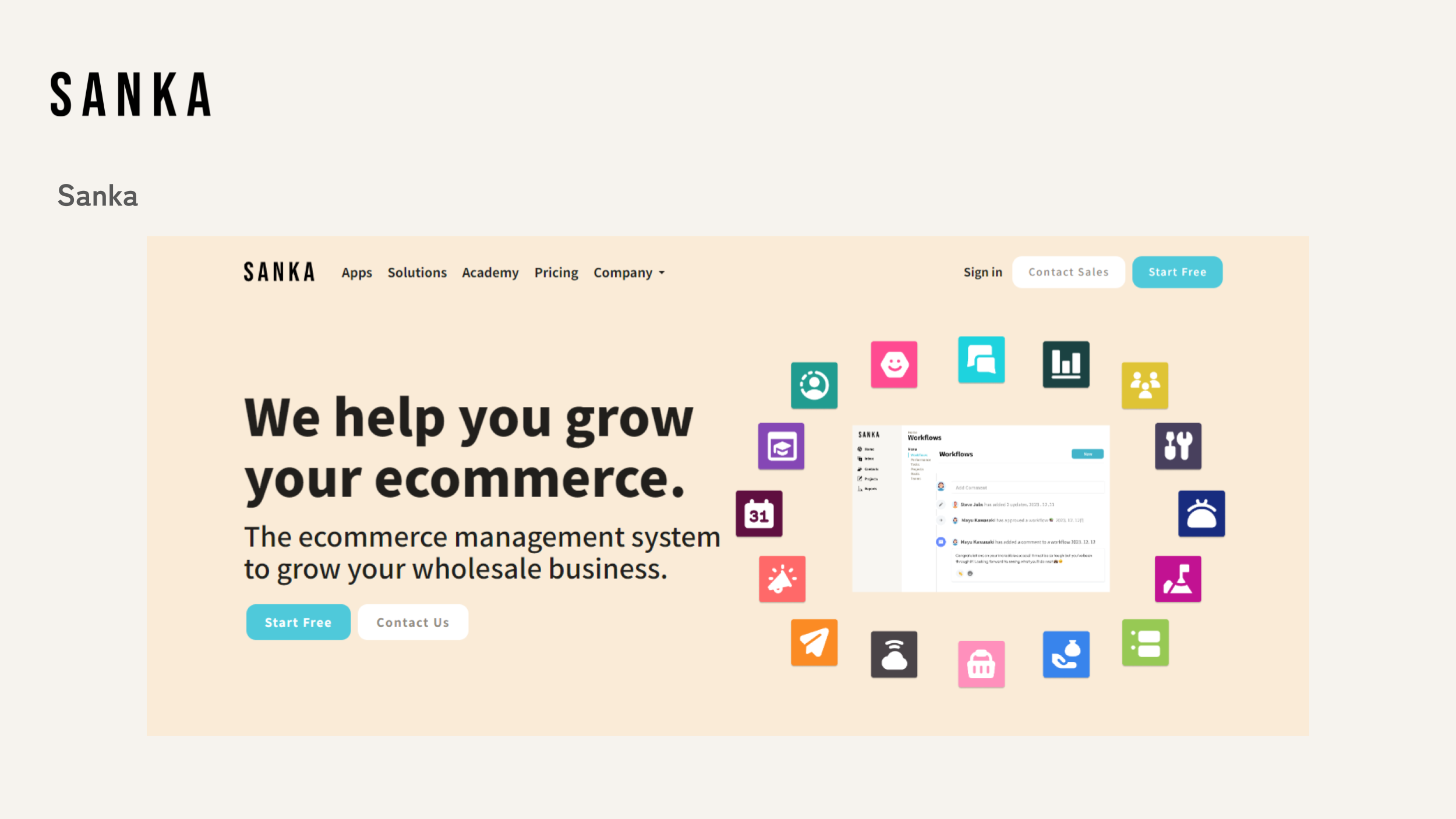The image depicts a web page with a light beige background, featuring a prominent central rectangular section in a brighter taupe shade. At the very top, the word "Sanka" is displayed twice in bold and regular fonts. Below this heading, within the taupe rectangle, are navigation elements: "Sanka," "Apps," "Solutions," "Academy," "Pricing," "Company," and a dropdown menu, with a "Sign In" option on the right-hand side.

Beneath the navigation bar, there is a white search bar accompanied by a blue "Start Free" button. To the left, a tagline reads, "We Help You Grow Your E-Commerce," followed by a brief explanatory sentence. Below the sentence, there are two buttons: a turquoise "Start Free" button and a white "Contact Us" button.

On the right side of this section, an illustration resembling a computer screen is displayed. The screen has a light gray left half and a white right half, featuring visible text. Surrounding the screen are various small square icons, each depicted in white against differently colored backgrounds, including a teal blue icon with conversation bubbles and a black icon with a bar graph, among several others, forming a circle around the illustration.